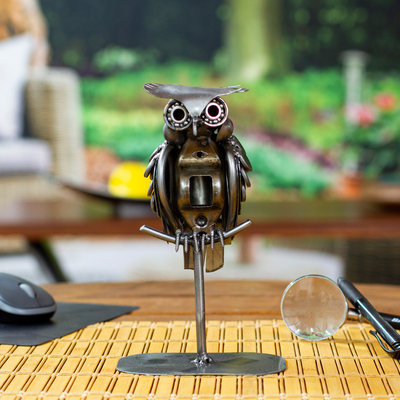The image features a minimalist metal owl figurine, centrally displayed on a small silver stand that resembles a jewelry holder. The owl is perched securely with its metal claws gripping the small divots on the horizontal bar of the stand. The entire setup is positioned on a light tan placemat, which rests on a wooden desk. To the left of the owl, there is a black mouse on a black mouse pad, while to the right, a black ink pen and a magnifying glass are easily visible. The blurred background suggests an outdoor scene with hints of a garden, showcasing purple flowers, green grass, and a tree. Additionally, part of a white wicker chair and another desk, possibly with a yellow object inside a black bowl, are faintly discernible.